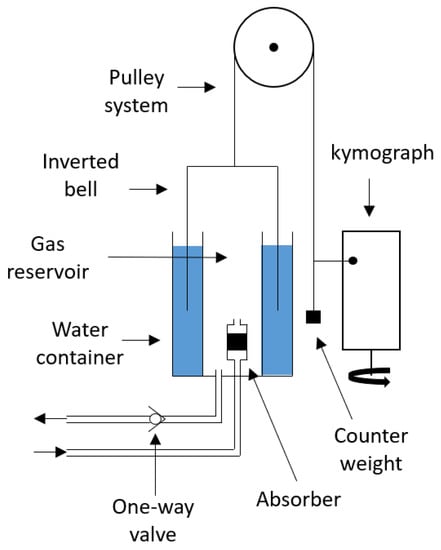The diagram presents a detailed schematic of an apparatus labeled as a 'chymograph'. Within a clean, white background, the various components and their relationships are meticulously depicted and clearly annotated with black text. At the top center of the schematic, a pulley system is illustrated, characterized by a circle with an attached pulley. 

To the left of the pulley, a line extends towards a vertical rectangle labeled 'inverted bell.' This rectangle houses an arrow leading to a section marked 'gas reservoir,' flanked by two smaller blue rectangles labeled 'water container.' From the base of this gas reservoir, two pipes enter with one leading to a component labeled 'absorber'.

On the right side of the pulley, another line descends to a small black square labeled 'counterweight.' Above this counterweight, a line extends further right to connect with another vertical rectangle, distinctly marked 'chymograph' in clear lettering. This rectangle stands on a small stand, resembling a vertical rectangle, indicating its position as the resultant output of the entire system.

Additional annotations in the diagram include 'one-way valve,' 'pulley system,' 'inverted bell,' 'gas reservoir,' 'water container,' 'absorber,' 'counterweight,' and 'chymograph,' clarifying the function and position of each element in this complex illustration. Despite the lack of an overarching title or frame, the diagram provides a structured and precise view of the interconnected apparatus, offering insight into the components and their roles within the system.